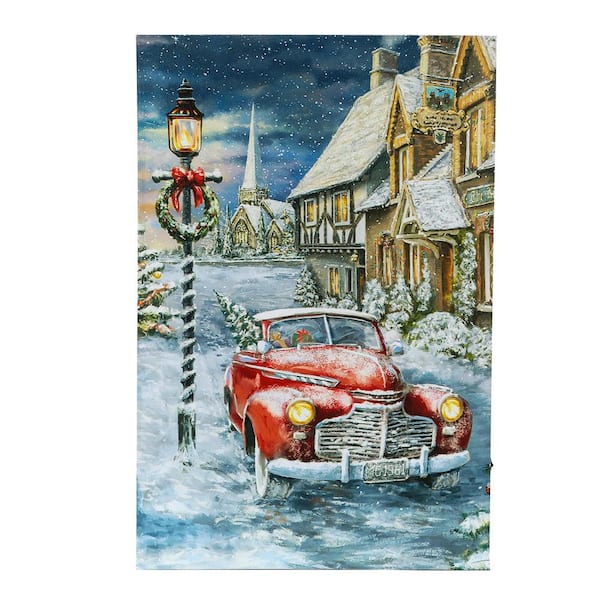The image depicts a picturesque, snowy night scene reminiscent of a classic Christmas card. In the foreground, a vintage red car, possibly a Chevy, is parked along a snow-covered road with its headlights facing the viewer. A Christmas tree is visible in the back seat, and presents are strewn across the passenger seat. Snow blankets the roofs and steeples of the buildings, adding a serene touch to the night. Dominating the background is a church with a tall steeple, also heavily laden with snow. Flanking the church are two old-fashioned English-style houses, one of which features a sign, hinting it might be a pub or tavern. A light pole adorned with a wreath wrapped in a red ribbon stands beside the car, adding to the festive atmosphere. The scene, depicted in portrait format, is set under a dark, snowy sky lit gently by the soft glow of street lamps, creating a warm and inviting holiday ambiance. The overall composition captures the charm and spirit of a tranquil Christmas night.